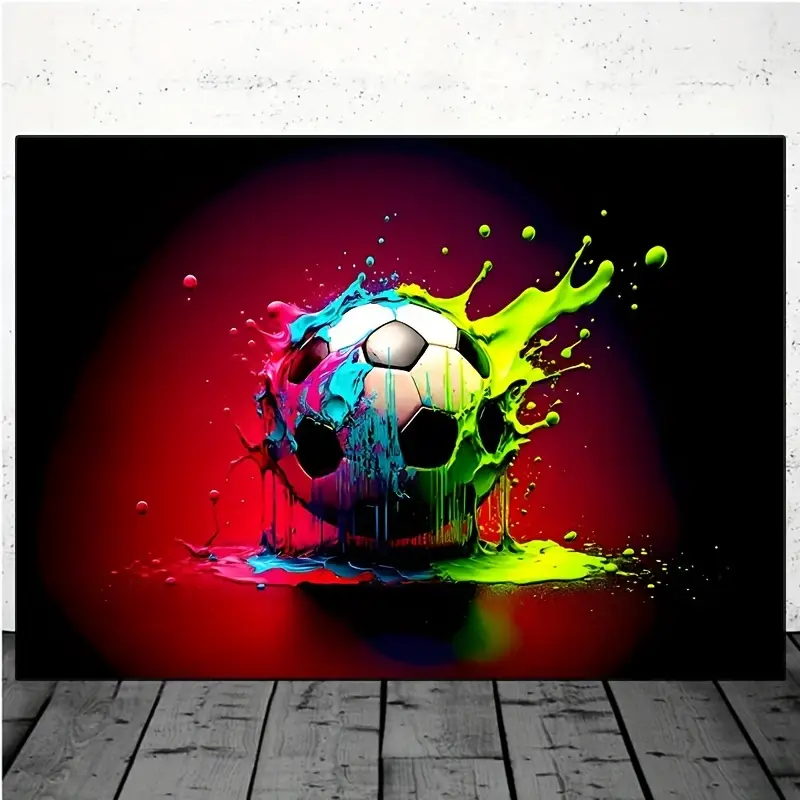The image is a detailed illustration of a soccer ball captured in a square-shaped poster. The poster takes up most of the image's width and leans against a white, speckled wall, partially visible at the top. Beneath the poster, vertical grayish-brown wooden boards with knots hint at a rustic floor. The borders of the poster are black, transitioning to bright red towards the center where the painted soccer ball is featured. The soccer ball, primarily black and white, is creatively splattered with vivid paint. Neon green splashes and drips down the right side into a puddle, while a blend of pink and blue paint cascades down the left, blending into another colorful puddle and splashing upwards. The scene captures the dynamic motion of paint droplets splattering around, emphasizing the vivid yellow, light green, light blue, pink, red, and purple hues. The poster appears to be photographed at eye level, leaning against the wall, with no additional text or words visible, suggesting an indoor setting.